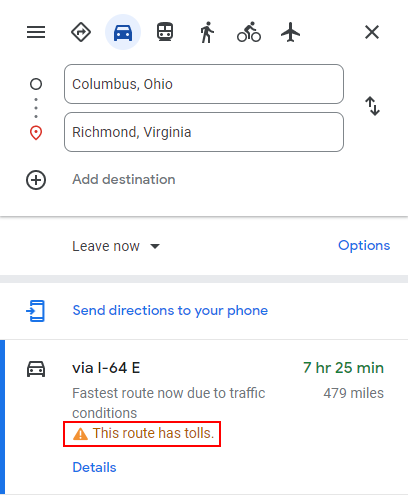The image depicts a detailed map application interface on a white background, designed to provide the best possible navigation routes between specified locations. At the top of the interface, a series of small icons and buttons offer various choices and settings. Starting from the left, there are three black horizontal bars, likely representing a menu for more options or settings. Following this is an icon for directions, depicted by a diamond sign with a direction arrow inside it. The highlighted car icon in blue indicates that the selected mode of transportation is by car. To the right of the car icon, sequentially, are icons for a trolley or bus, a person walking, a person on a bike, and finally, an airplane, each representing different transportation options.

In the upper right corner, a gray X serves as a close or cancel button. Below this top menu, the screen displays the journey details, starting from Columbus, Ohio, and heading to Richmond, Virginia. There is an option to "Add destination" with a plus sign, and another option labeled "Leave now," both of which are clickable for further customization. Additionally, there is a clickable blue link labeled "Adding directions to your phone."

The route is specified as via I-64E, which is the fastest route. It notes that due to traffic conditions, this route includes tolls and estimates a travel time of 7 hours and 25 minutes, covering a distance of 479 miles. Further details about the route are available below this information.